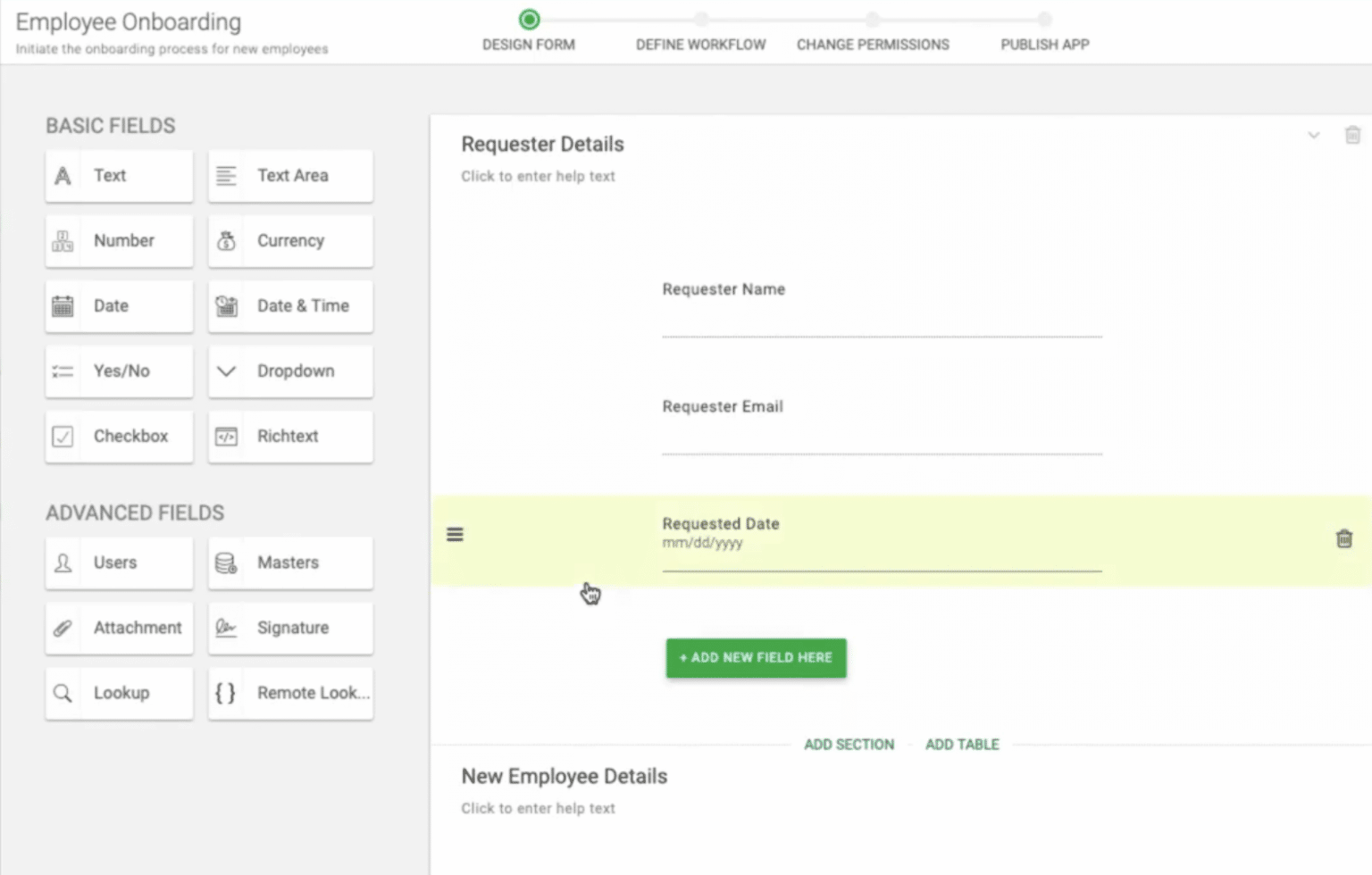The image illustrates an employee onboarding process for an employer. On the left side, there's a section with a white background and black text titled "Employee On-Boarding." Below this title, there is some smaller, unreadable text, with the last two words being "new employees." A horizontal bar indicates the current stage in the process. Directly below the bar, the steps are listed as: Design Form, Define Workflow, Change Permissions, and Publish App.

In a gray box on the left side labeled "Basic Fields," there is a 2x5 grid with white rectangles and black text containing the following fields: Text, Text Area, Number, Currency, Date, Date and Time, Yes/No, Drop-Down, Checkbox, and Rich Text.

Another section underneath is labeled "Advanced Fields," arranged in a 2x3 grid with entries for Users, Masters, Attachment, Signature, Lookup, and Remote Lookup.

In the main part of the image, there's a large white area with black text that reads "Request Your Details" and "Click to Enter Help Text." Following this, the fields are listed as Register Name, Register Email, with a highlighted orange section marked "Requisition Date: MM/DD/YYYY."

In a green box with white text, there are options to "+ Add New Field Here," "Add Section," and "Add Table." Finally, underneath, there's a directive for "New Employee Details" with an option to "Click Here to Enter Help Text."